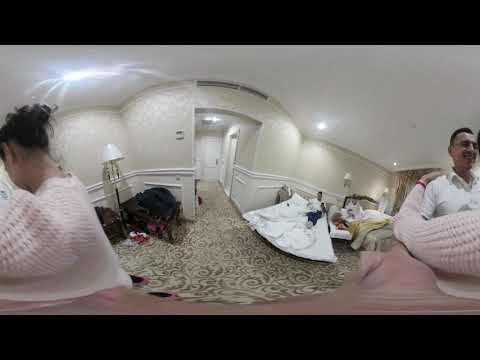In this heavily distorted 360-degree photograph of an indoor room, likely a hotel room or a bedroom, we see a blend of intriguing elements due to the wraparound effect. The floor is covered in a patterned carpet, and the walls are painted a soft eggshell cream color with white crown molding along the bottom. 

The room also features a bed with a black frame and yellow sheets positioned on the right. There's another bed next to it, separated by a nightstand. A large white blanket lies on the floor next to the bed, with someone laying on it and partially out of view. 

Taking center stage in the photograph is a man with lighter skin, dressed in a black and white polo shirt. His right arm, holding the camera, is noticeably distorted, stretching towards the bottom edge of the image. Just beyond him, there's a woman captured twice in the photograph, a result of the 360-degree effect. She appears on both the right and left edges of the image. 

The woman, identifiable by her black hair tied up and her soft pink cable-knit sweater, has her left arm wrapped around the man's right shoulder. The back of her head faces the camera on the left edge of the photo. The entire scene is framed by a white ceiling and includes a small hallway leading to a door, completing the layout of this surreal, immersive image.